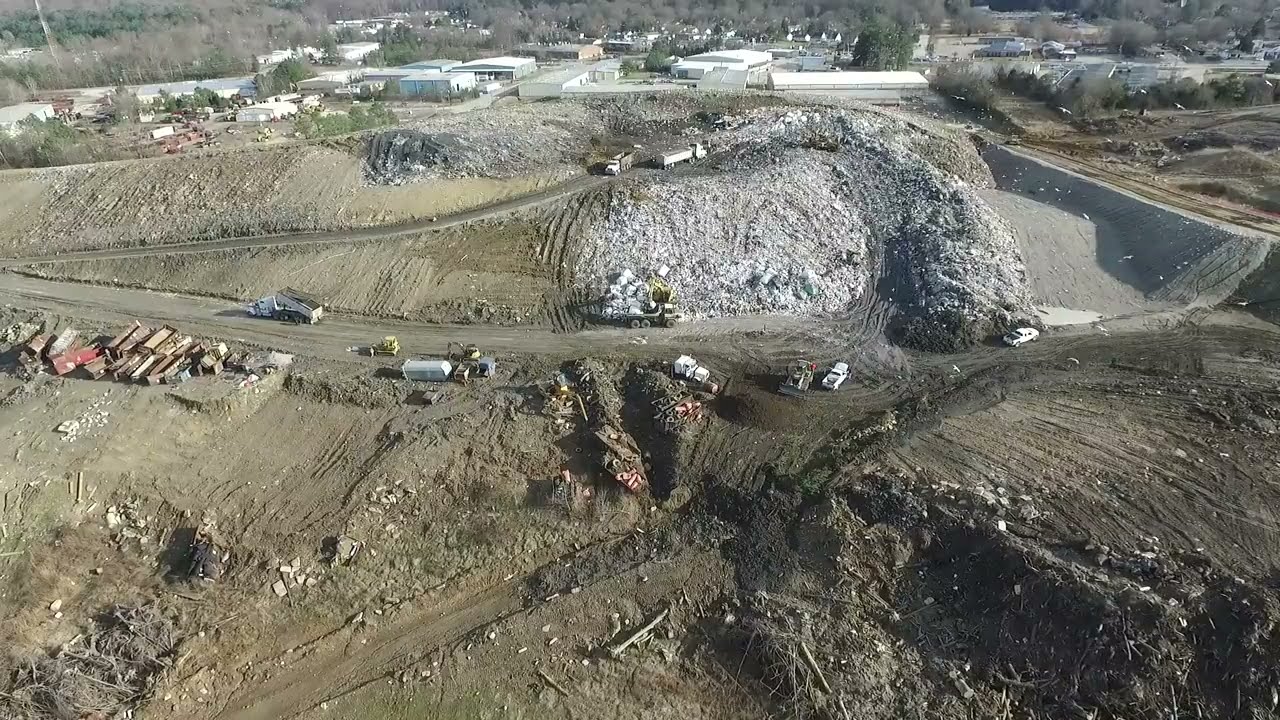The image captures a sprawling construction site characterized by a rocky, worn terrain with a lot of exposed soil and boulders scattered throughout. Prominent in the center is a hill composed of gray gravel. Surrounding the gravel hill is a dirt road, extending both around and through the site, which appears to have been recently paved, evidenced by the soil being moved. Various construction trucks—including dump trucks, diesel semi-trucks, and pickup trucks—are dispersed throughout the area, some parked on the road and others seemingly in operation.

In the background, the construction site extends to an industrial area filled with white warehouse buildings of different shapes, including long rectangles and square structures. Distant trees frame the industrial zone, giving a sense of depth to the landscape. Additionally, the image hints at the possibility of dam construction on the right-hand side, where there's a sloping, concrete-filled area. The perspective appears to be aerial, offering a comprehensive view of the bustling site, with some storage boxes visible on the left-hand side, possibly storing equipment or materials for the ongoing construction activities.